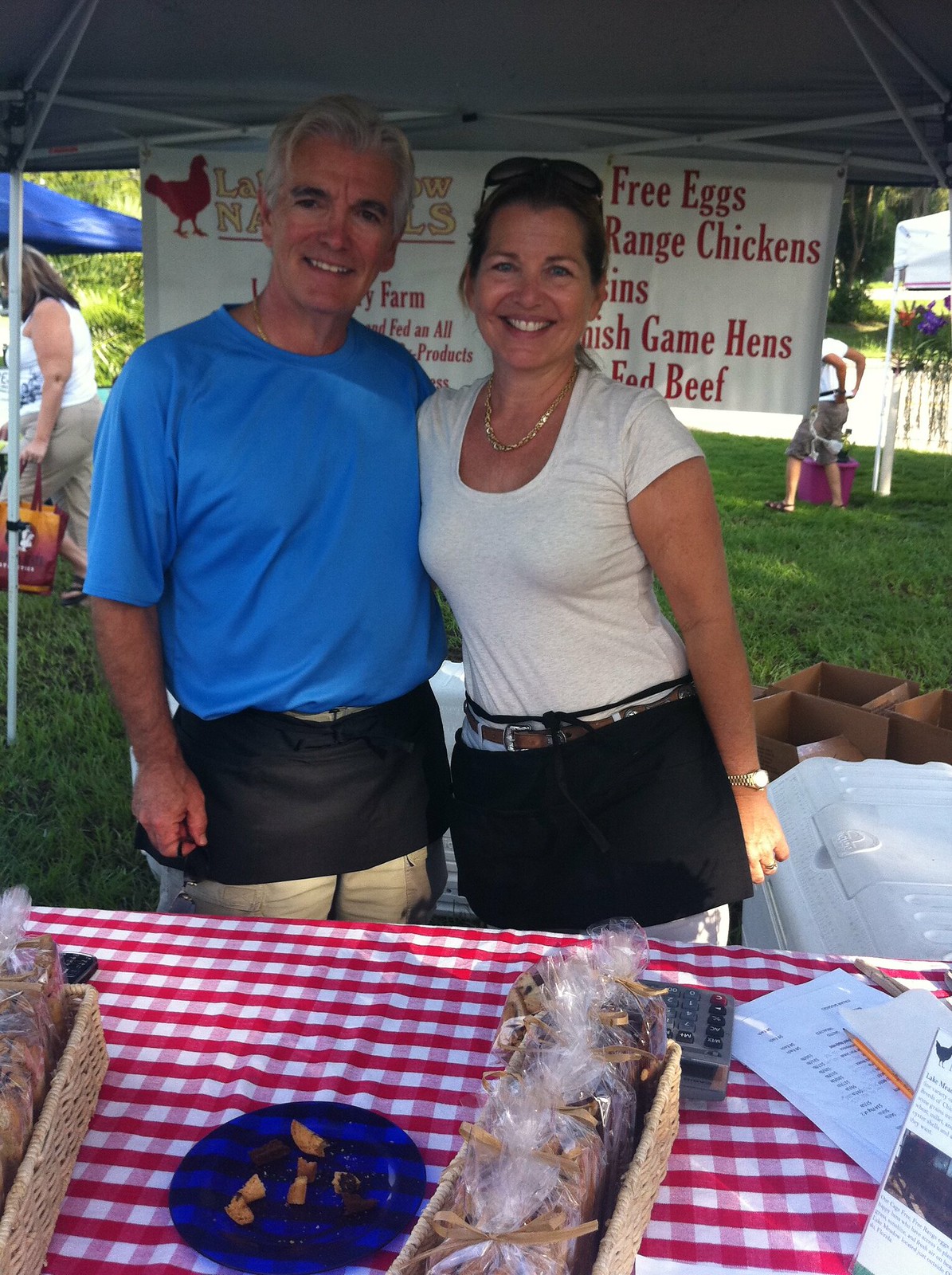A man and a woman are pictured at a market stall, standing in front of a table covered with a red and white checkerboard tablecloth. The table holds a blue plate with food, cellophane-wrapped baskets tied with gold bows, a calculator, and some pieces of paper. The man, on the left, is smiling and wearing a blue shirt, gray hair, black eyebrows, shorts, and a small black apron around his waist. The woman, on the right, is also smiling, dressed in a white T-shirt, a gold necklace, sunglasses on her head, a small watch, an apron around her waist, and a belt. They are under a canopy, with signs in the background including a white one with red text that reads "Free Range Chickens, Free Eggs, Game Hens Fed Beef," accompanied by a red chicken icon. The background features a grassy area, more people, and additional market stalls.